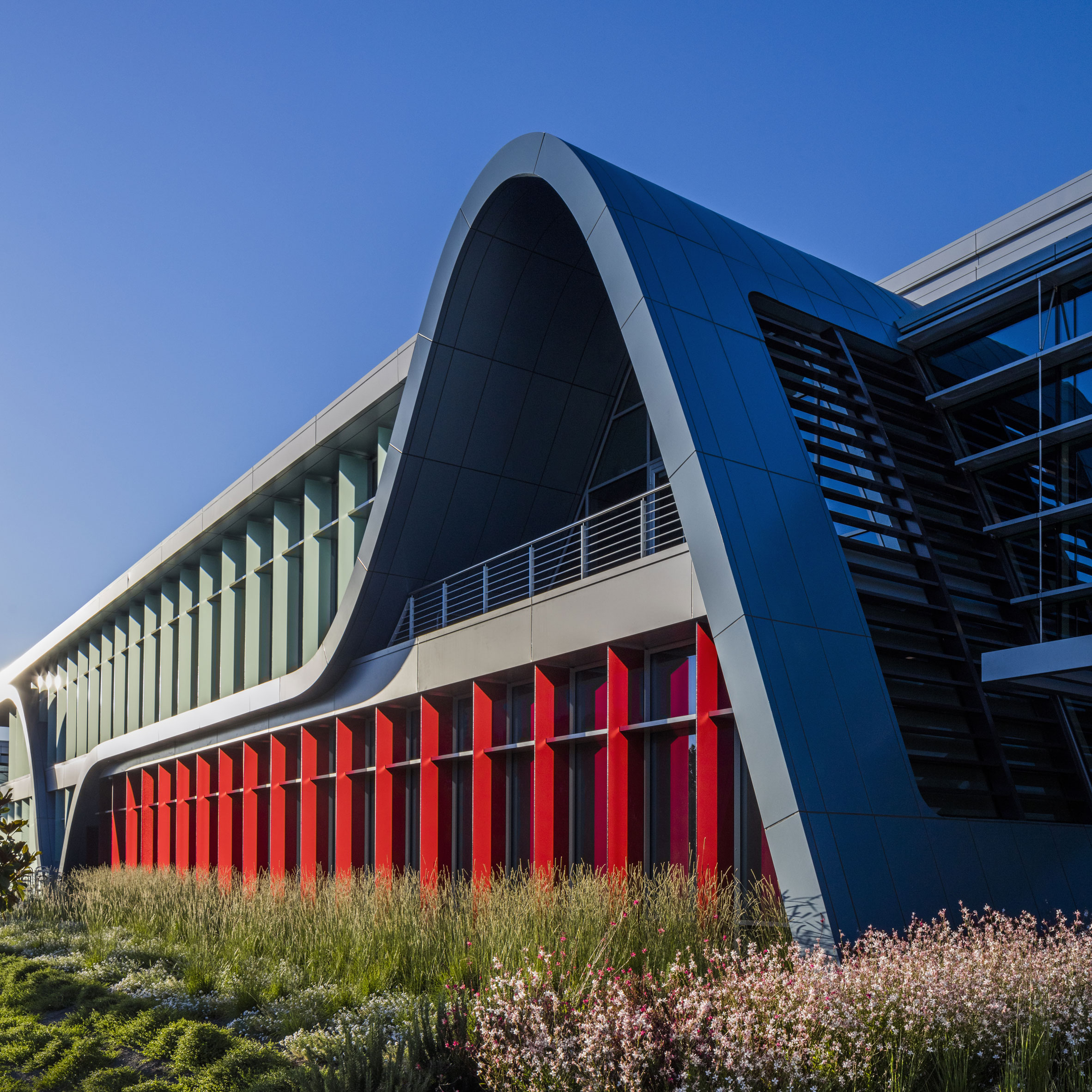This photograph, taken outdoors on a clear daytime, features a modern, wavy-styled building set against a blue sky. At the bottom of the image, there's a variety of tall grasses, weeds, and wildflowers, including some with small white blooms on the right side. The building boasts a series of red windows on the ground level, transitioning to gray windows on the second story. A notable architectural feature is the wavy arch with fins that allows airflow, and a deck with a railing. To the left, additional windows display a similar design, and in the upper right, a large expanse of windows connects to the central wave structure, contributing to the building's contemporary aesthetic.